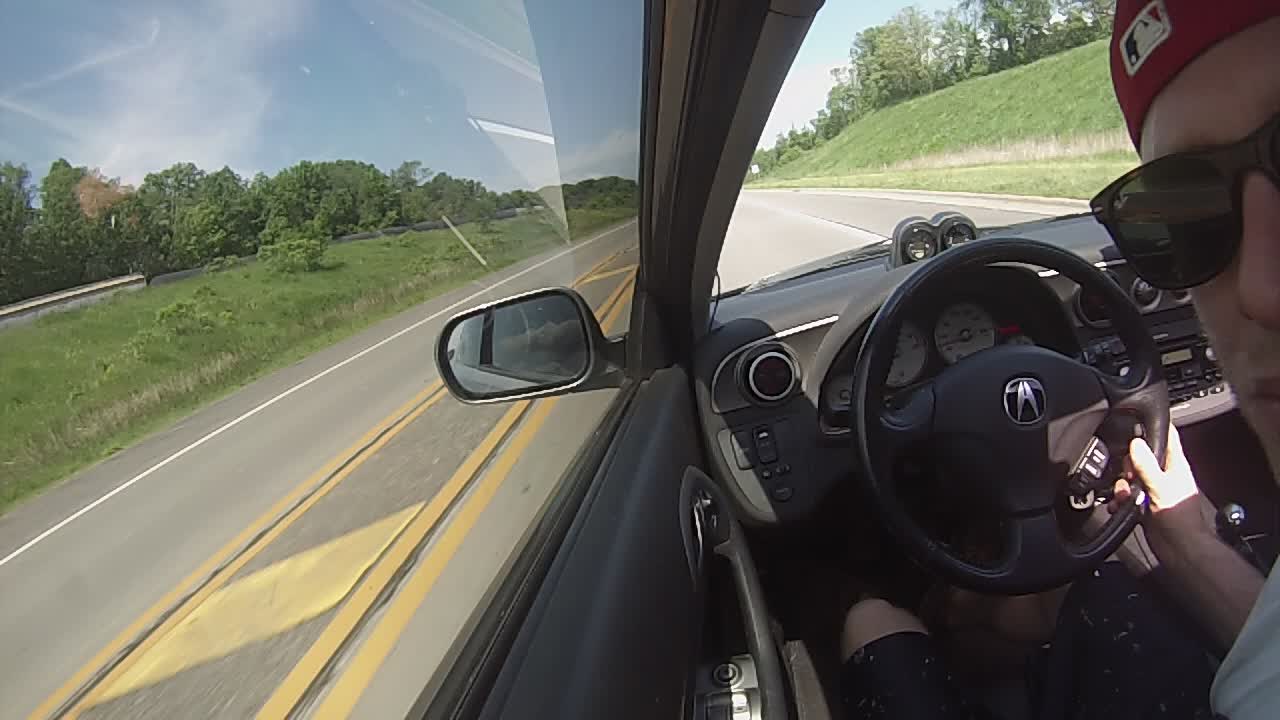The image depicts a driver in a later model car, likely a Kira, on a clear day driving on a highway. The driver, who is wearing black shorts and a red baseball cap with the Major League Baseball logo on backwards, is looking back at the camera while holding the black steering wheel with his right hand. He's also wearing sunglasses. The photograph appears to be a selfie, with the driver using his left hand to position the camera behind his right shoulder, though it could also be taken by someone else seated behind him. Visible within the car are tinted windows, appearing somewhat dim inside despite the bright, clear day outside. The interior of the car looks clean and well-maintained. Through the windows, you can see the highway's lanes, including an HOV lane marked by yellow dotted lines, and the surrounding landscape featuring grassy hills and green bushes on either side of the road. The sky is a vivid blue, indicating a perfect driving condition.